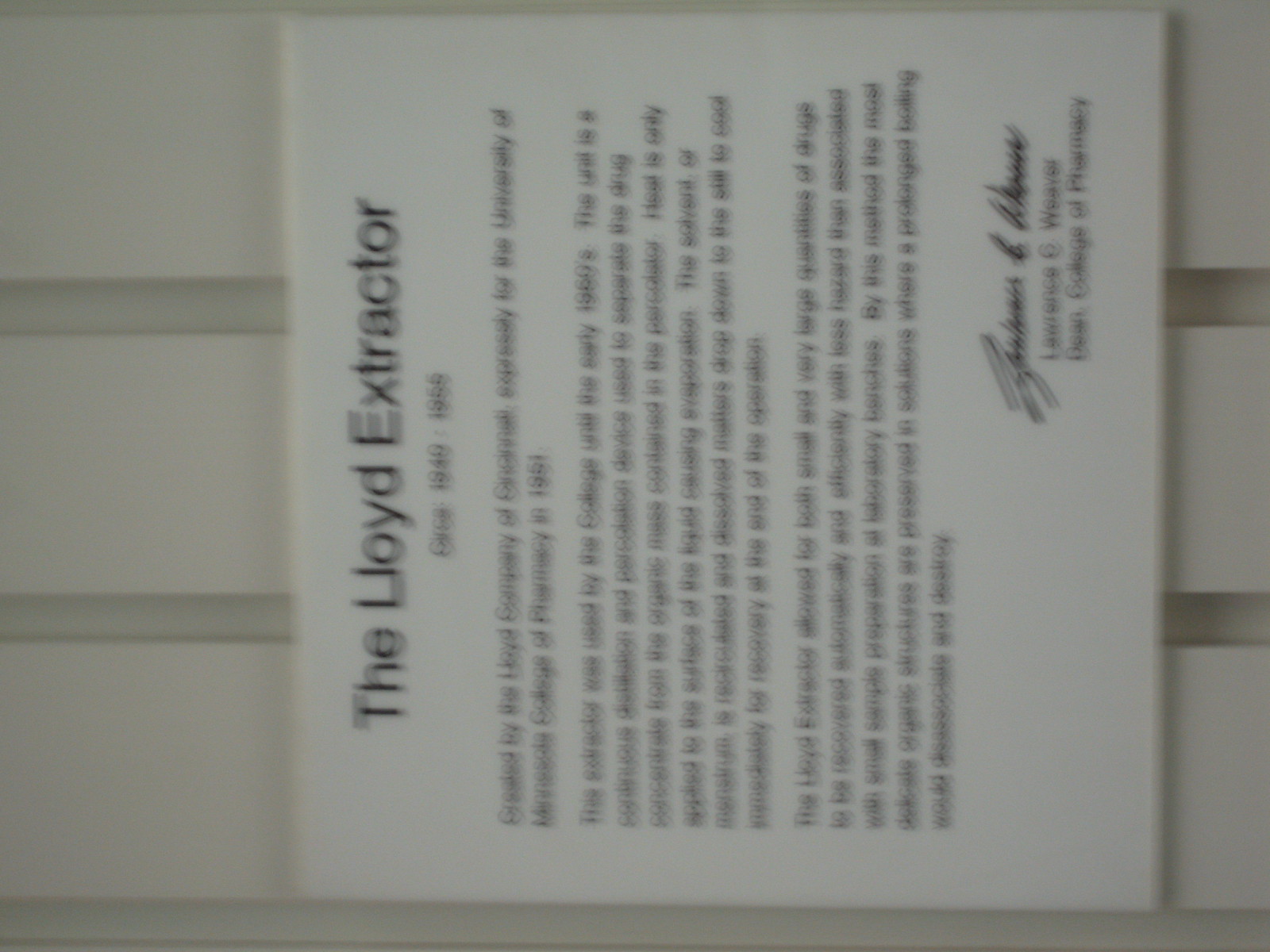This image features a rectangular sign hanging on a wall, captured from a side angle, making the text appear slightly skewed. The background is a gray surface that resembles wall siding. The sign itself, resembling a sheet of paper, bears black text. At the top, a prominent header reads "The Lloyd Extractor." Beneath the header, in smaller font, is a date range that appears to be "1940 to 1955" or perhaps "1940 to 1956." Following the date, there are several paragraphs of smaller, largely illegible text. The document concludes with a signature, followed by the inscription "Lawrence G. Weaver, Dean, College of Pharmacy."